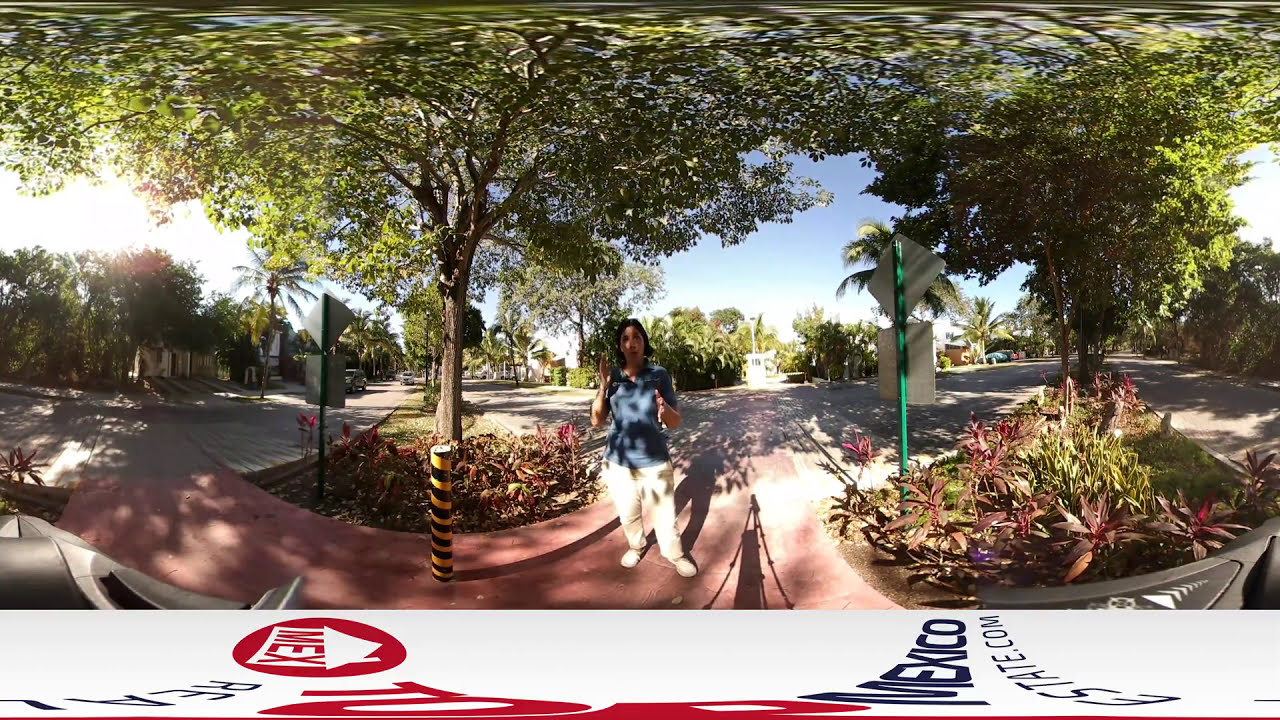The image is a daytime, landscape-oriented photograph, likely taken with a fisheye or panoramic lens that has caused a distorted, stretched effect. At the center of the image stands a person, possibly a woman, wearing a blue shirt and white or khaki pants. She has medium-length dark hair and appears to be holding something in her left hand while looking directly at the camera, as if explaining something. The surrounding area features a walkway that curves and continues both behind and in front of her. To the left of the walkway, a street originates from the image's left side and curves away, bordered by houses and trees. To the right of her, a sidewalk stretches from the bottom right and moves away into the distance, flanked by trees or bushes. An area of dirt, grass, a tree, flowers, and other bushes is situated in the foreground, with another street visible on the far right side. The bottom of the photograph includes a white border with stretched-out, hard-to-read red and blue writing, including the word "Mexico" on the right. The overall scene appears to be in a suburban area with diverse foliage, possibly in Mexico, as suggested by the visible text and the presence of a palm tree. The sky is blue, and the sun's position to the back left creates dappled shadows and patches of direct sunlight.